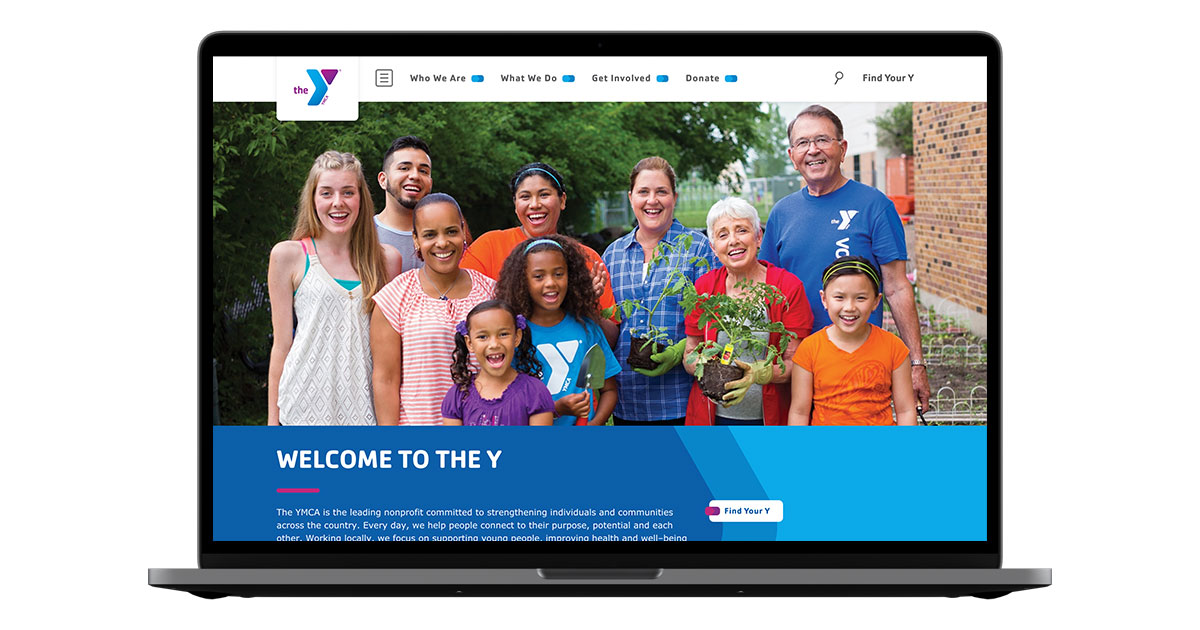A screenshot captures a laptop screen with a black top and bottom border displaying a welcoming message for the Y. The central part of the screen features a diverse group of people, each individually identifiable by their distinctive clothing. From left to right, the image showcases a girl in a white dress, a man in a gray shirt, a woman in a pink shirt with white stripes, a woman in an orange shirt, and a girl in a blue shirt sporting a white logo. Additionally, there is a girl in a purple shirt, a girl in a plaid blue shirt holding a plant while wearing green gloves, an older woman with white hair in a red coat and gray shirt holding a plant, a man in a blue shirt, and a little girl in an orange shirt. The screen's upper portion prominently announces "Welcome to the Y" in black text, while the bottom section features additional information in white text.